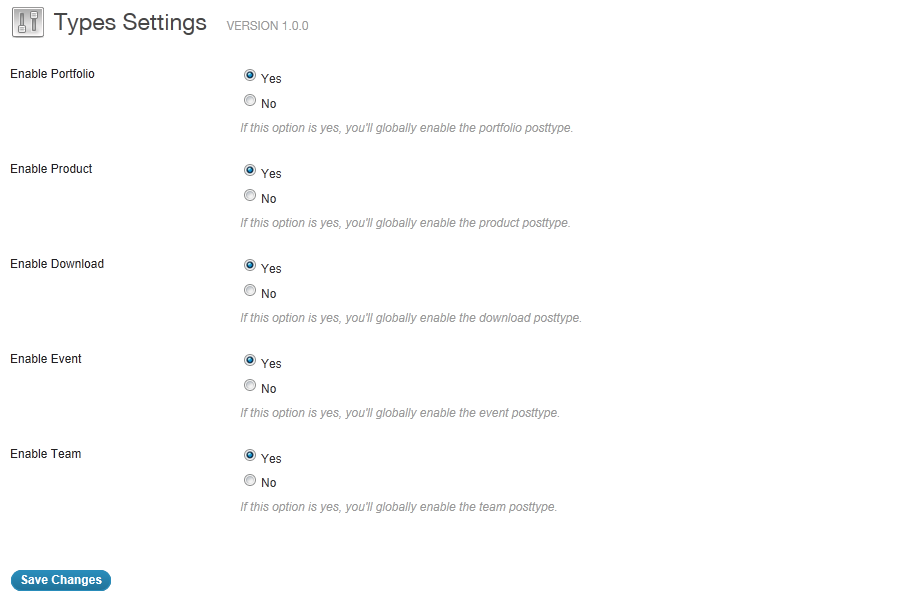The image showcases a settings interface with a white background. In the top-left corner, there is a small blue box featuring two spatula-like icons—one oriented upright and the other upside down. The header of the interface reads "Type Settings Version 1.0.0". Below the header, there are several setting options presented in a checklist format:

1. **Enable Portfolio:**
   - **Yes** (selected with a blue dot)
   - **No**
   If the "Yes" option is selected, this setting will globally enable the "Portfolio" post type.

2. **Enable Product:**
   - **Yes** (selected)
   - **No**
   If the "Yes" option is selected, this setting will globally enable the "Product" post type.

3. **Enable Event:**
   - **Yes** (selected)
   - **No**
   If the "Yes" option is selected, this setting will globally enable the "Event" post type.

4. **Enable Team:**
   - **Yes** (selected)
   - **No**
   If the "Yes" option is selected, this setting will globally enable the "Team" post type.

At the bottom of the interface, there is a prominent blue button labeled "Save Changes". All the options for enabling portfolio, product, event, and team post types are checked "Yes", indicating they are all activated.